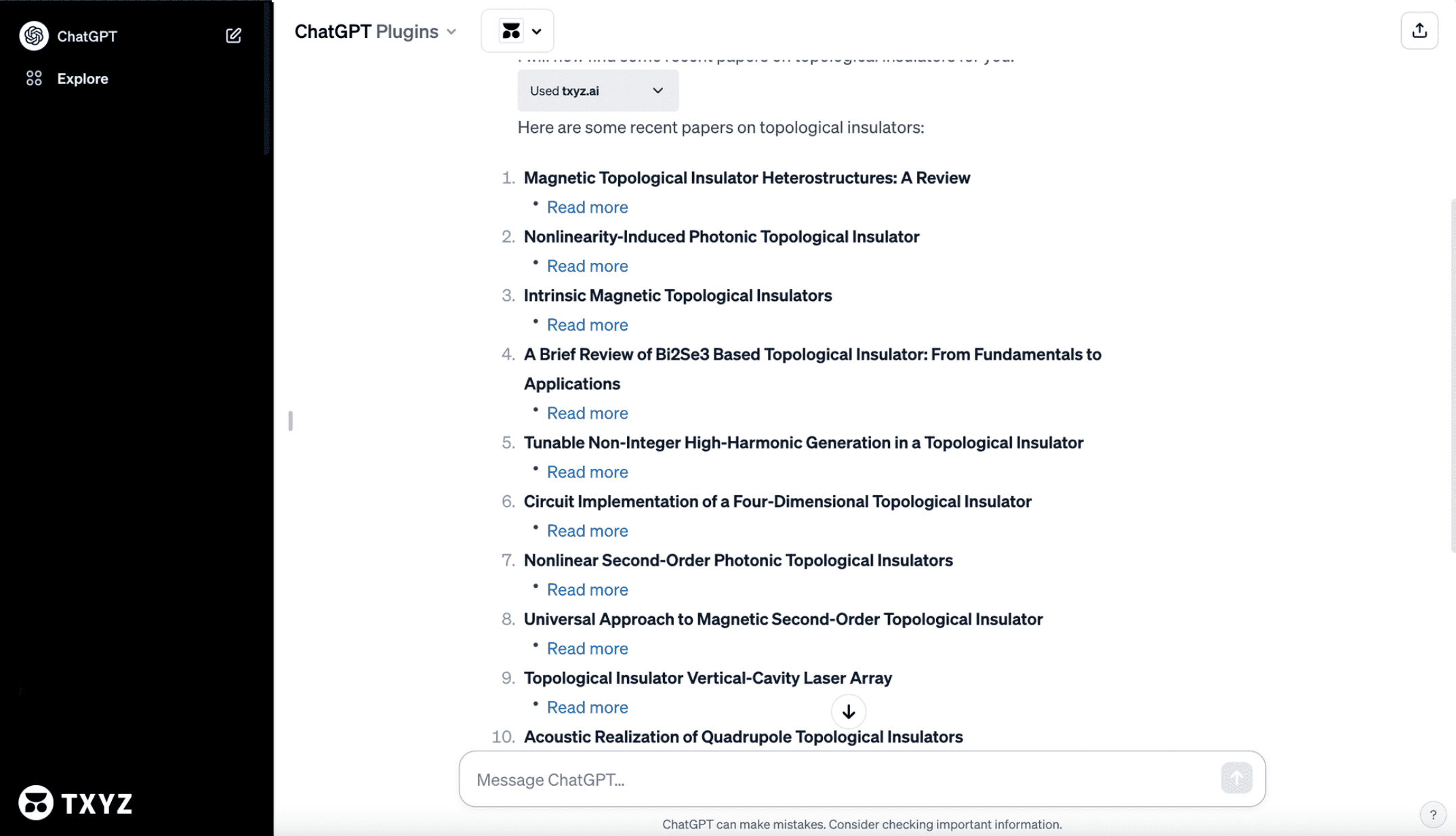The image is a screenshot of the ChatGPT interface in use. On the far left, there is a black vertical rectangle featuring the ChatGPT logo, which resembles a line-drawn rose. Next to the logo, the text "ChatGPT" is displayed in clear, bold letters. Below this section, there is a square icon with a pencil in its corner, indicating an editable feature, and beside it are four dots (two at the top and two at the bottom) with a label that reads "Explore."

Additionally, a small semicircle icon is visible with its round edge facing downward. Flanking this icon are two smaller circles, and adjacent to it are the letters "T-X-Y-Z." The central part of the screen is predominantly white, and it displays a header that reads "ChatGPT Plugins." Below this header, there is a chat box where the text "Message ChatGPT" is visible, indicating the input area for user interaction.

In the conversation thread, the AI has provided a response that mentions "Here are some recent papers on topological insulators," followed by a list of titles such as "Magnetic Topological Insulator Heterostructure: A Review," and "Magnet Topological Insulators," among others. The information indicates that the AI is being queried for scholarly references related to topological insulators, demonstrating its capability to retrieve and present academic papers on the topic.